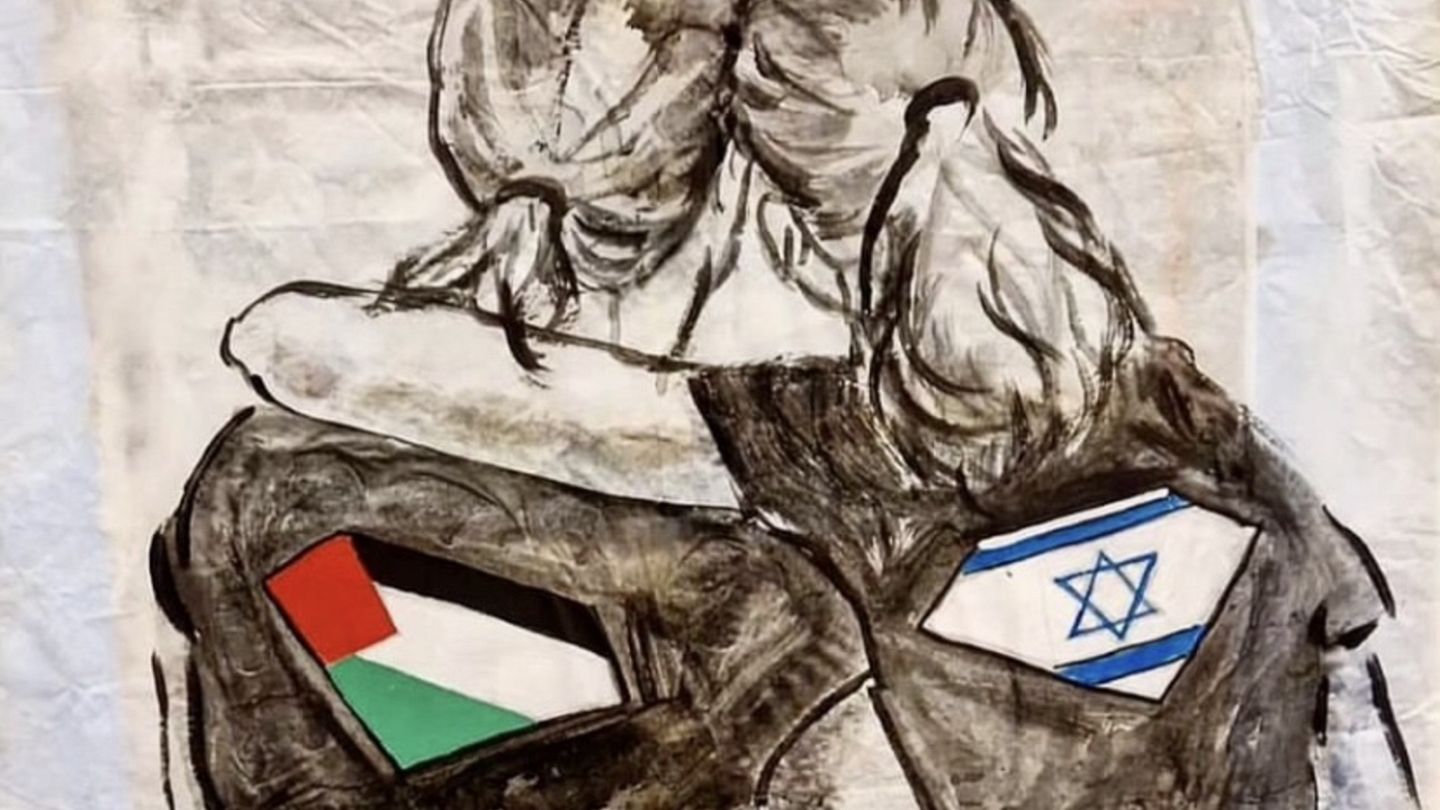This detailed black-and-white pencil sketch captures two people, presumed to be a man and a woman, in an intimate embrace, viewed from behind. The man, on the left, has shorter hair tied in a ponytail and is distinguished by his left arm and shorter shirt sleeves. The woman, on the right, sports a longer ponytail and has her left arm lovingly draped around the man's neck. Both their shirts prominently feature diamond-shaped symbols on the back, each representing different flags: the Palestinian flag on the man's shirt, with its distinctive black, white, and green stripes alongside a red square, and the Israeli flag on the woman's shirt, characterized by blue stripes at the top and bottom with a blue Star of David in the center. The sketch, while predominantly monochromatic, subtly incorporates mild browns and colored elements for the flags, enhancing the emotional gravity of the depiction. The background texture resembles wrinkled fabric in beige and white hues, adding depth. Overall, the artwork poignantly conveys a message of unity and reconciliation between the two nations.